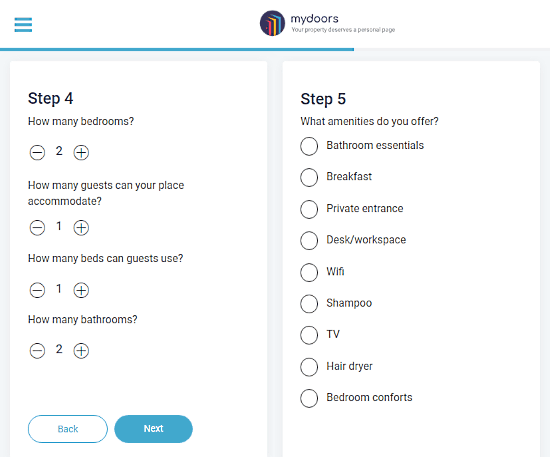The image depicts a user interface for listing a property on a rental website. In the top left corner, there is a section marked by lines, while a circle, colored sections in red, yellow, and blue, appear near a door icon which is identified as "my door" on the property. Below, the interface includes a personal page with a blue bar highlighting "Step Four".

Several input fields are presented:

1. "How many bedrooms?" with options to adjust the number using minus and plus signs.
2. "How many guests can your place accommodate?" with similar plus and minus adjustment options.
3. "How many beds can guests use?" with minus and plus options.
4. "How many bathrooms?" also adjustable with minus and plus signs.

Additionally, an oval labeled "back" and another blue oval with white text reading "next" are present. Below is "Step Five" asking, "What amenities do you offer?" with the following options listed but not selected:
- Bathroom essentials
- Breakfast
- Private entrance
- Desk or workspace
- Wi-Fi
- Shampoo
- TV
- Toilet paper
- Clothes dryer
- Bedroom comforts

The background of the page is grey. On the right side, there is a vertical series of 9 circles, colored and laid out in a sequence.